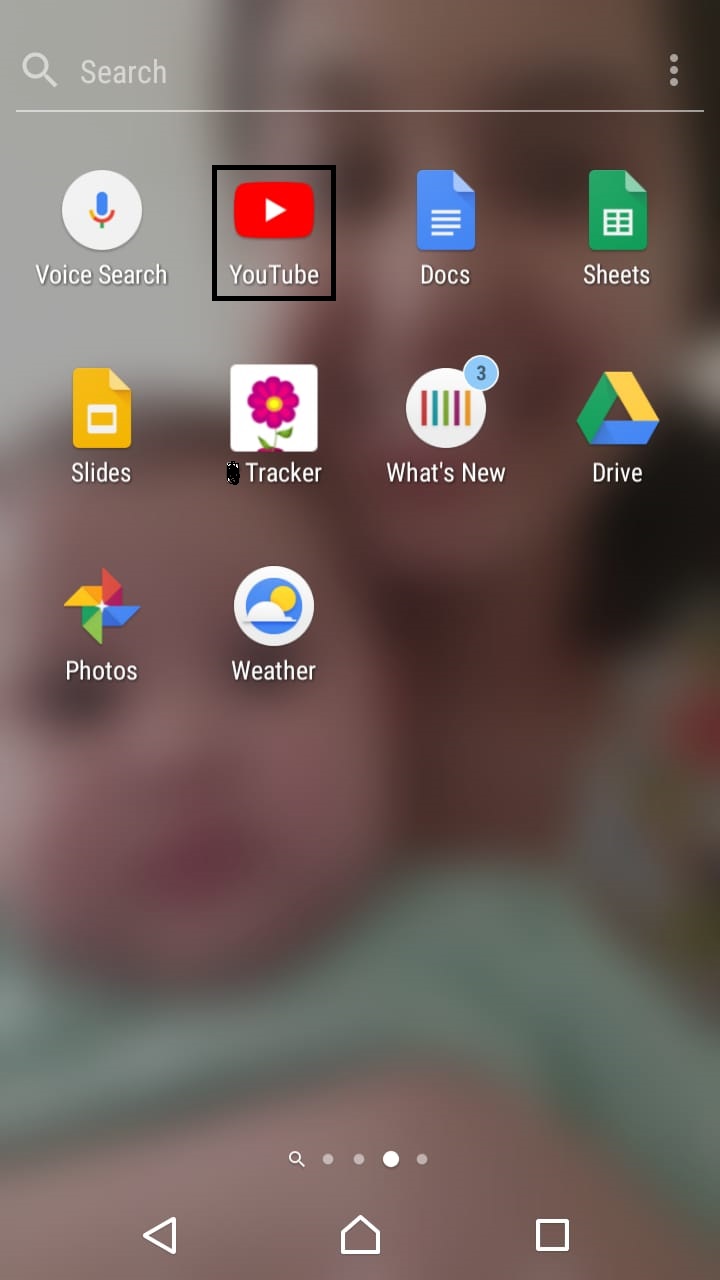The image depicts a user interface screen divided into multiple sections. 

At the very top, there is a magnifying glass icon followed by a search bar containing the word "Search." To the far right of this top section are three vertical dots indicating additional options.

Beneath this, the screen is organized into three distinct rows of icons:

1. **First Row (left to right):**
   - **Voice Search Icon**
   - **YouTube Icon**, which is distinctive with a black box surrounding it
   - **Three Dots Icon**
   - **Heat Icon**

2. **Second Row (left to right):**
   - **Slides Icon**
   - **Tracker Icon**
   - **What's New Icon** with three notifications indicated
   - **Dry Icon**

3. **Third Row (left to right):**
   - **Photos Icon**
   - **Weather Icon**

Below the rows of icons, there is a pagination indicator showing that this is the third page out of four. The indicator consists of:
- A magnifying glass symbol for the first page
- Two dots representing the second and third pages
- The third dot is highlighted, indicating the current page
- The fourth dot is gray, signifying a non-active page

At the very bottom of the screen, there's a navigation bar featuring:
- **Play Button** to the left
- **Home Button** in the center
- **White Square Button** towards the right

This detailed layout provides clear navigation and functionality cues for the user.